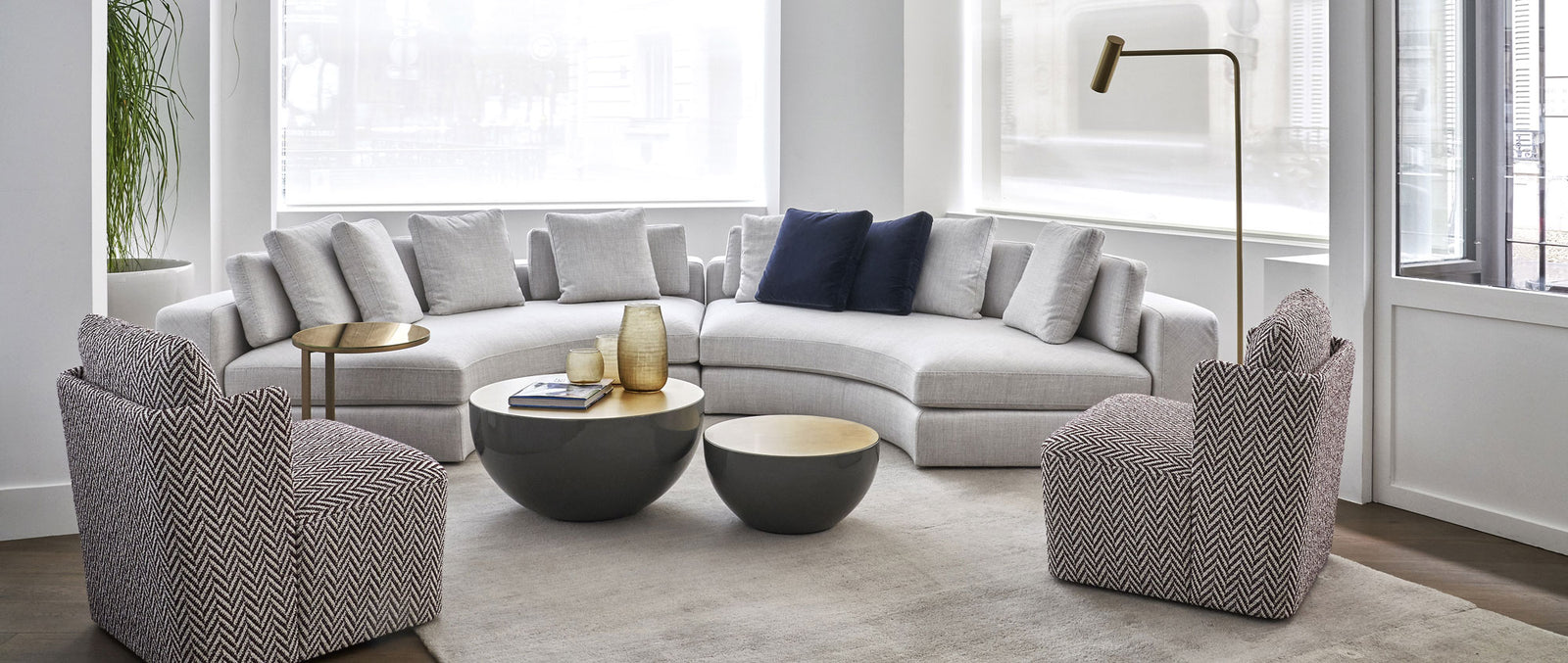This picture features a chic and modern living room bathed in natural light from its large, white-painted walls and expansive windows. The focal point is a large, crescent-shaped white sectional sofa, which is divided into two main sections, each capable of seating two or three people. The sofa is adorned with an assortment of white pillows and two dark navy accent pillows. Flanking the sofa are two cushioned chairs, showcasing a sophisticated brown and white herringbone pattern. A substantial, pristine white rug grounds the space and enhances the room's monochrome elegance.

In the center of the seating area are two distinctive coffee tables made from two different-sized green half-globes with flat wooden surfaces. One table features a collection of three empty glass vases in varying shades of yellow and a book, while the other holds a pitcher and some glasses. The room includes tasteful decor elements such as a large green plant in a white pot located in the top left corner, a stylish lamp, and subtle gold accents that add a touch of luxury. The brown wooden flooring further underscores the contemporary, yet comfortable aesthetic of this sophisticated living room landscape.